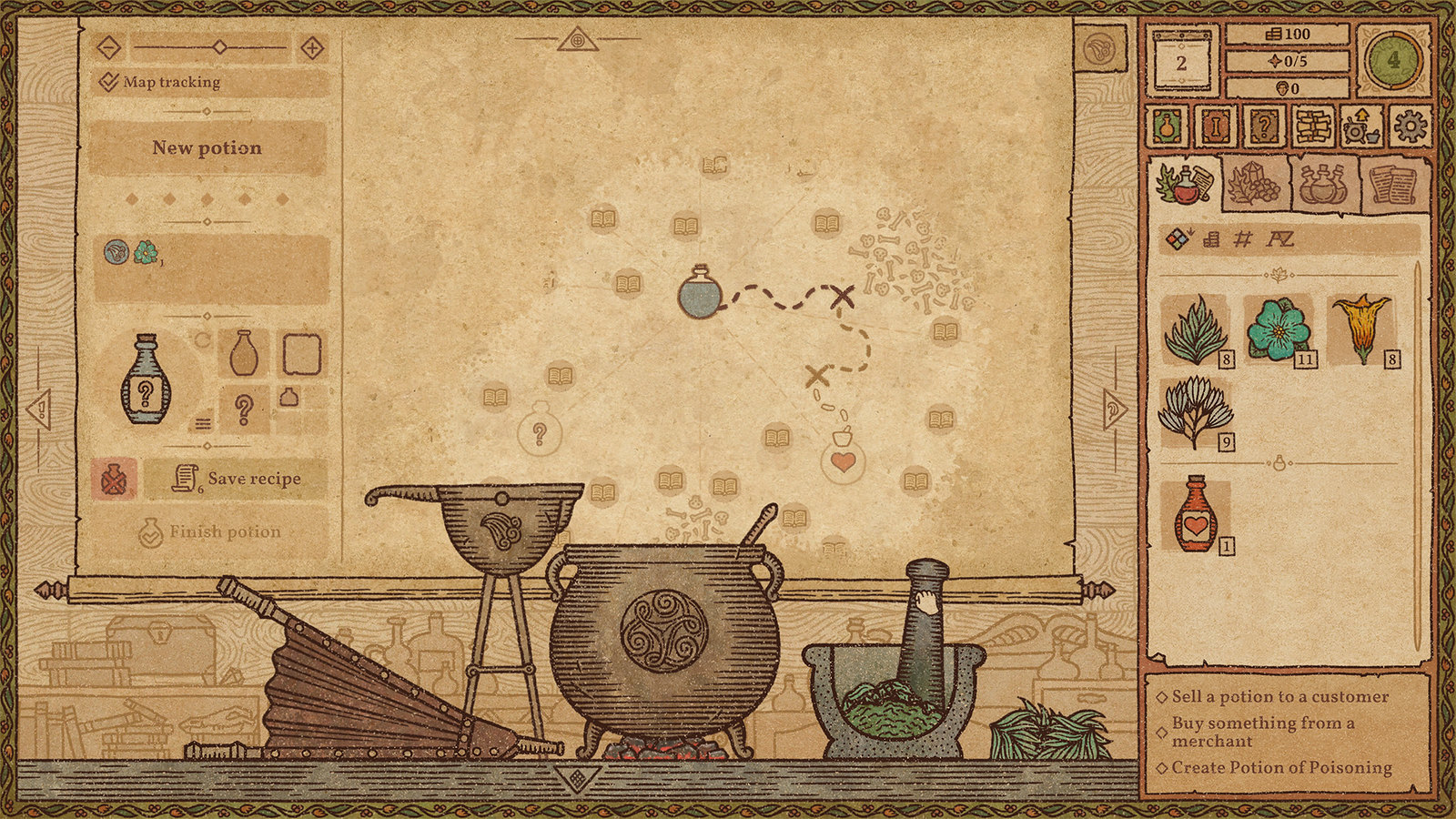The image portrays a screenshot from an older-style video game with an illustrated, vintage visual aesthetic, dominated by brown, tan, and green hues. Central to the image is a map labeled "map tracking" in the top left corner, ensconced in a scroll-like display, resembling old-school roll-down screens found in classrooms. The illustration also features a detailed setup for creating potions, including various cauldrons, bottles, and a mortar and pestle. Key elements such as "new potion," "save recipe," and instructions like "sell a potion to a customer," "buy something from a merchant," and "create potion of poisoning" are prominently displayed. The potion bottles vary in appearance, with notable details like a blue bottle marked with a question mark and another bottle with a red X. Decorative items, including what appears to be herbs, flowers, and fireplace implements, add to the rustic, hunter-gatherer vibe of the scene.